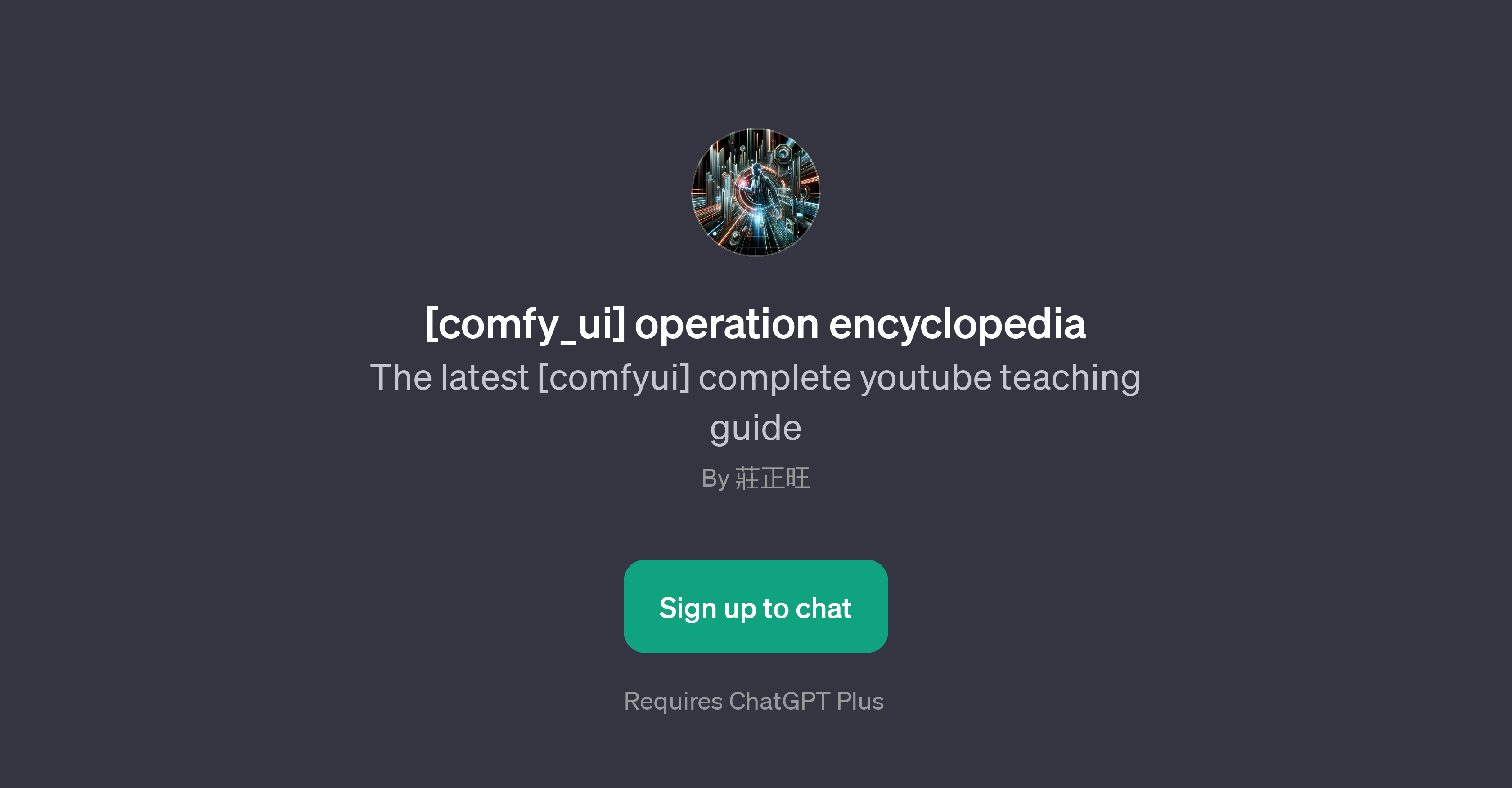In this rectangular screenshot with a dark gray background, we have a horizontally extended layout featuring a prominent, centrally positioned, round disc reminiscent of a vinyl record. The disc's design prominently features a primarily black surface adorned with subtle rays of blue, white, and pink radiating from its center, contributing to a visually appealing contrast. Below the disc, in bold white text, the caption reads "comfy_UI_operation_encyclopedia." Directly underneath, in subtler gray text, the descriptive phrase "The latest Comfy_UI complete YouTube teaching guide" is displayed. Further down, a vibrant green action button is prominently placed, featuring the call-to-action "Sign Up to Chat" in white text. Finally, a note below the button indicates, "Requires ChatGPT Plus," implying the need for a premium subscription to access the feature.